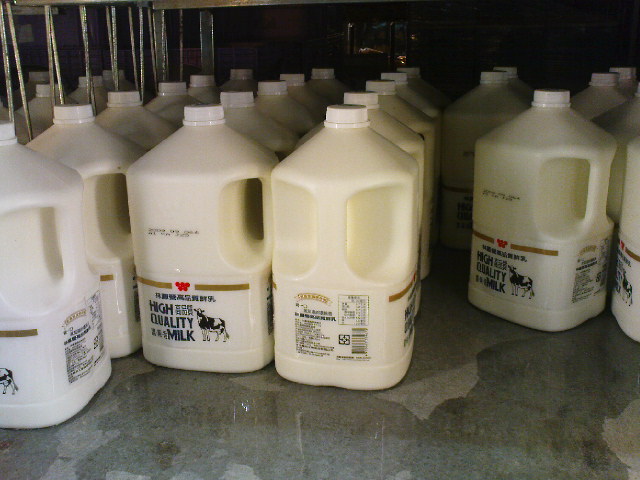The image depicts numerous rectangular cartons of milk arranged in several distinct rows on what appears to be a concrete floor, indicating a possible setting within a factory or a manufacturing plant rather than a grocery store. The environment suggests the milk is being prepared for transport, perhaps loaded onto a truck. Each milk carton features a white label with black text, including branding that reads "high quality milk" alongside a picture of a cow. The labels incorporate Asian characters, likely providing details such as expiration dates to ensure freshness. Additionally, the packaging displays a red logo with a gold stripe, nutritional information, and a barcode. The ground beneath the cartons appears wet in several areas, adding to the industrial feel of the setting.